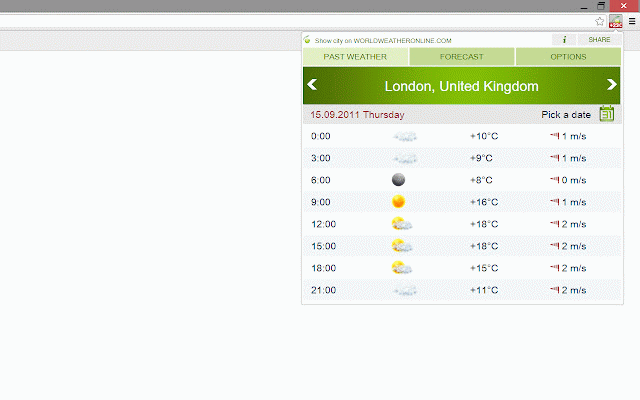The image depicts a weather forecast website focused on providing historical weather data for London, United Kingdom. At the top of the page, there are three primary functions: "Past Weather," "Forecast," and "Options," with the "Past Weather" function currently active. Beneath this menu, the location is prominently displayed as "London, England," flanked by left and right arrows, suggesting the ability to navigate between different pre-set cities.

Below the location, the current time and date are shown, accompanied by a calendar feature that allows users to select any past date for which they want to view weather data. The main section of the webpage features a detailed table with four columns: 

1. **Time:** Lists various times of the day, segmented into three-hour intervals starting from midnight (00:00, 03:00, 06:00, 09:00, 12:00, 15:00, 18:00, 21:00).
2. **Weather Icons:** Displays small images representing the weather conditions at each time slot (e.g., cloudy, sunny, partly cloudy).
3. **Temperature:** Indicates the temperature in Celsius for each corresponding time.
4. **Wind Speed:** Presumably shows wind speed in miles per hour for each time interval.

There are about ten rows in total, providing a comprehensive hourly breakdown of the weather conditions for the selected date.